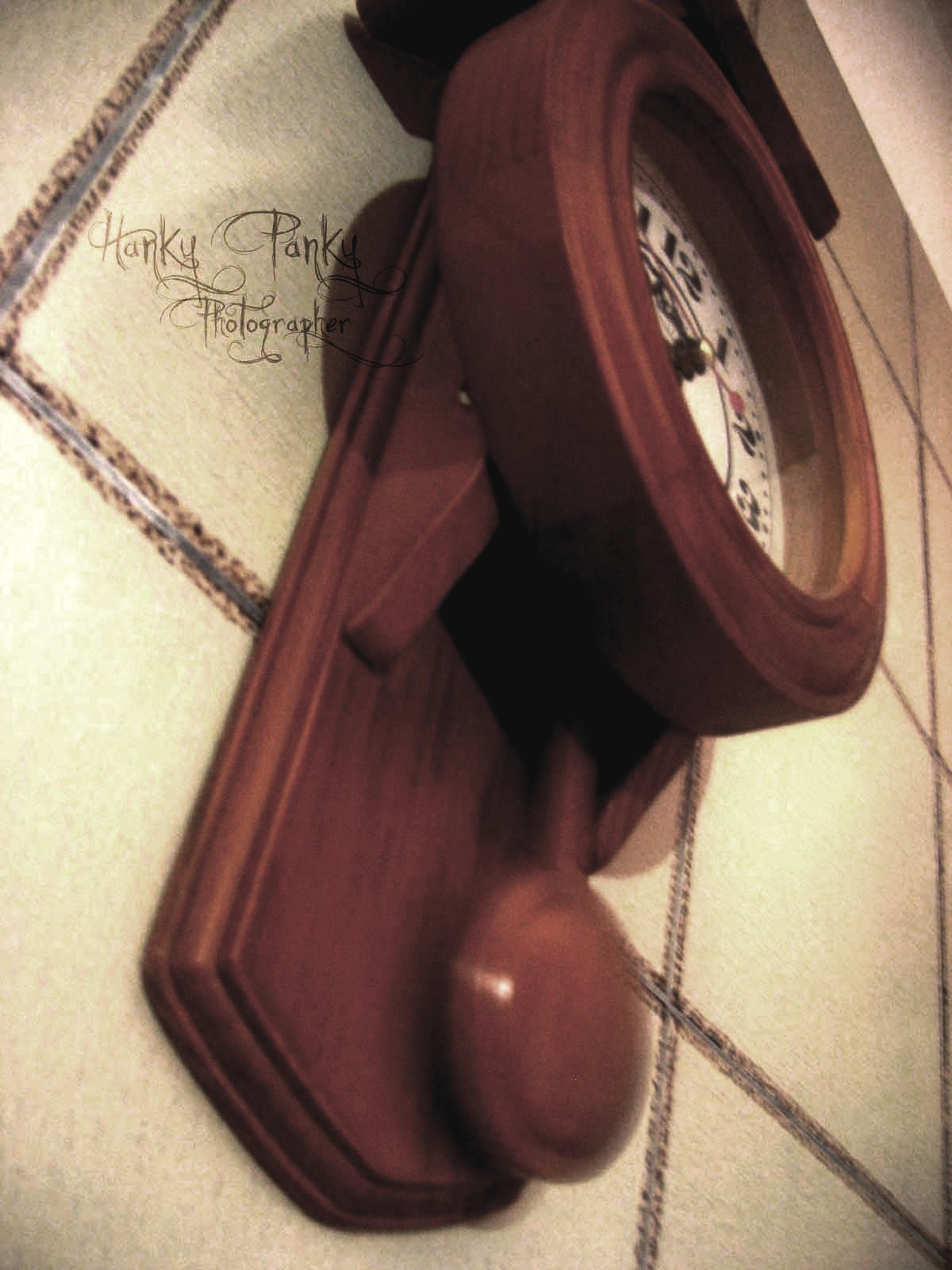This is a photo taken from an upward perspective of a vintage wall clock. The clock features a thick, circular wooden outer frame that partially obscures the white clock face from this vantage point. The face itself is adorned with black numbers and dots marking the minutes, while black metal hands indicate the time. Mounted on a medium brown wooden board, the clock adds a classic touch with a pendulum hanging just below the face, which is captured in a blurred state, indicating motion. The clock is fixed on a wall covered with white tiles interspersed with green and brown grout, creating a striking contrast. In the upper left-hand corner of the image, the words "Hanky-Panky Photographer" are handwritten in elegant, flowing script.